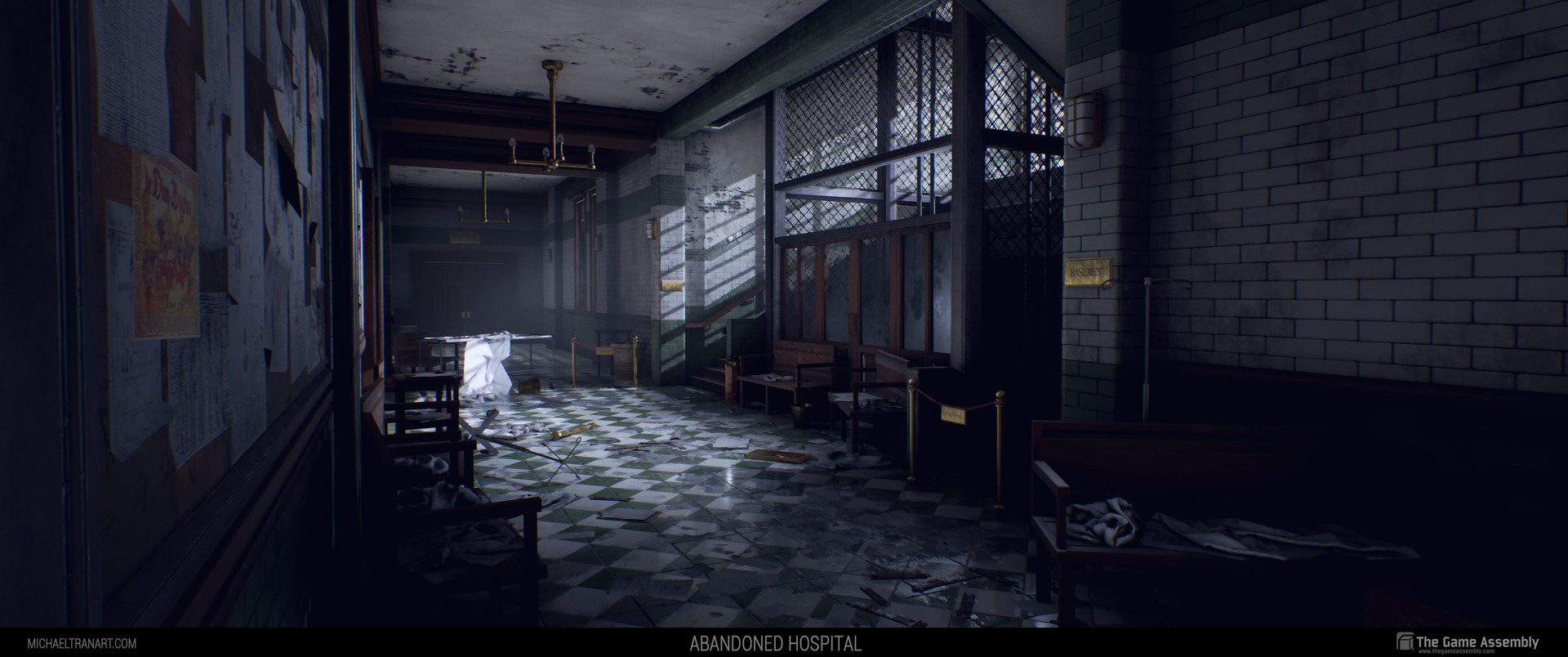This image, likely a highly realistic rendering from a video game, shows the eerie interior of an abandoned hospital hallway, as indicated by the text at the bottom reading "Abandoned Hospital" and "MichaelTranArt.com" on the left with "The Game Assembly" in the bottom right alongside a website. The floor is a checkerboard pattern of green and white tiles, strewn with debris and various pieces of furniture, emphasizing the deserted nature of the scene. To the left, a bulletin board is cluttered with mostly white papers, featuring a distinct golden yellow sheet among them. The hallway is shrouded in darkness, except for some light filtering in through a high window on the right, casting shadows that hint at the barred windows and glass panes below it with wooden frames. On the opposite side, brown doors and white brick walls with a brass light fixture hanging from the ceiling can be discerned, while a golden sign, possibly indicating "Basement," adds to the desolate atmosphere. The detailed mess and scattered placements contribute to the overall feel of abandonment, resembling a school-like environment but distinctly marked as a hospital.